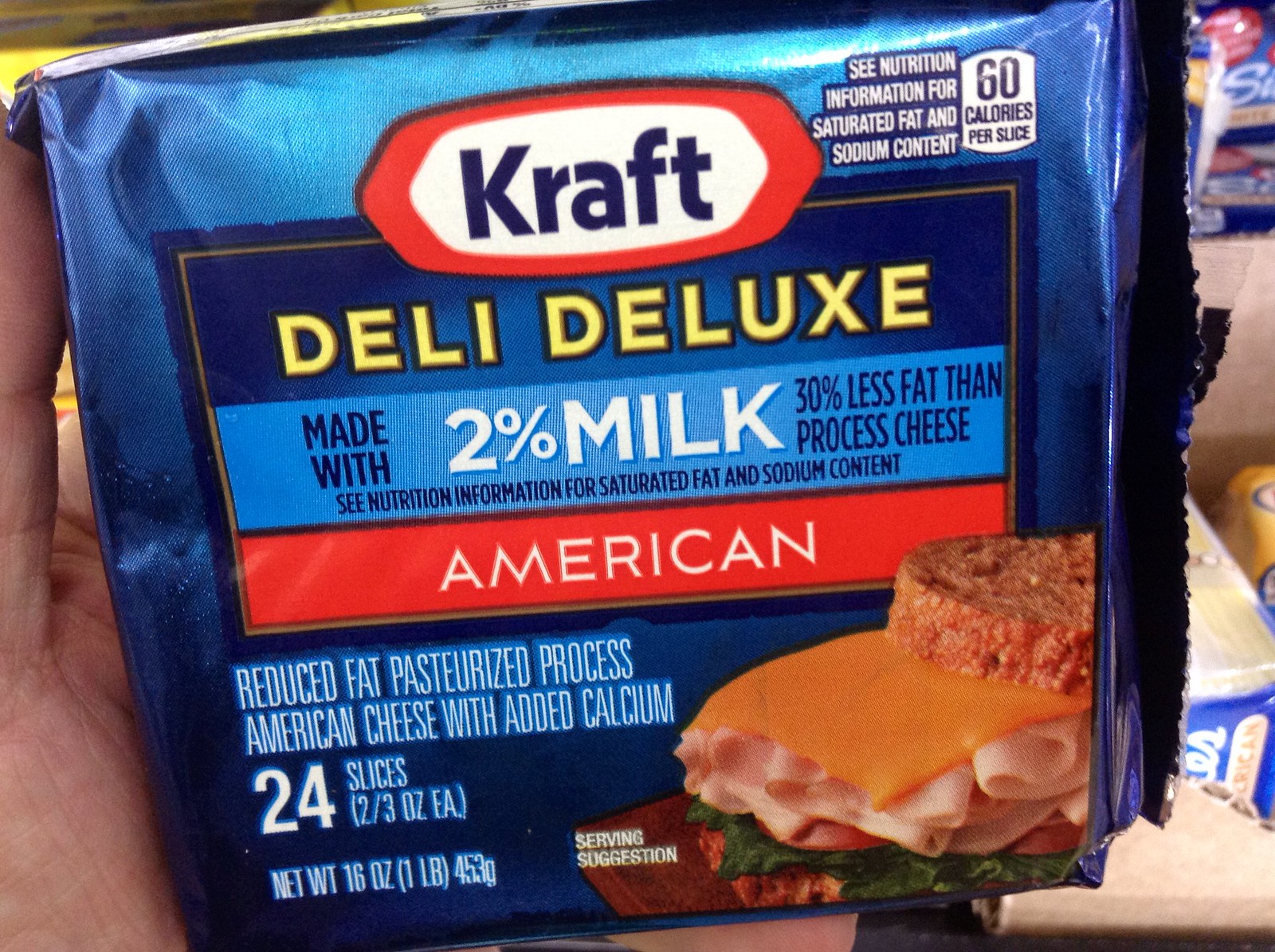This square image prominently displays a blue package held by someone's hand on the left side. Taking up most of the frame, the package features detailed labeling. The top right corner states, "See Nutrition Information for Saturated Fat and Sodium Content." Additionally, "60 calories per slice" is printed nearby. At the top center of the packaging, the brand name "KRAFT" is displayed, followed by "Deli Deluxe." Below this, the text notes, "Made with 2% milk, 30% less fat than processed cheese." The image underscores the nutritional details and branding of this cheese product.